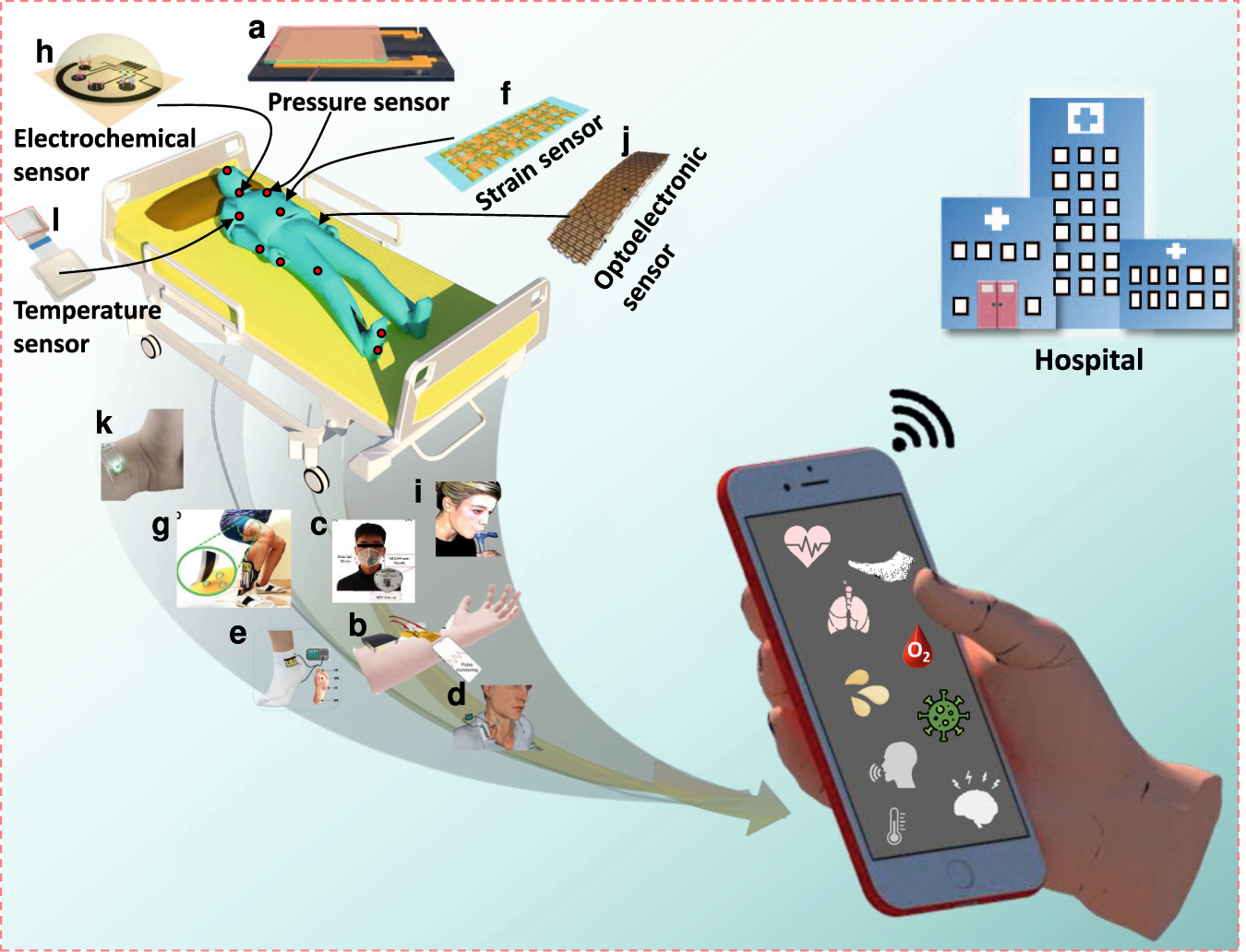The image depicts a digital alert system for hospital trips integrated with a smartphone. In the foreground, there's a hand holding a cell phone, showing a gray background on the screen with diagrams representing various health indicators, including heart, water, germs, cough, head injury, and temperature. The phone has a blue front and a red outline on the back. Surrounding this central element, on the left side and top, are various medical diagrams and sensors—pressure, electrochemical, temperature, strain, and optoelectronic—connected to different regions of a blue-colored human figure lying on a silver bed with a red cover. Arrows from these sensors point towards the smartphone, indicating a data flow. Below the bed, a large arrow, initially as wide as the bed, thins as it extends downward and rightward, also pointing towards the smartphone, symbolizing the transfer of information. In the background, on the right side, there's an image of a blue hospital complex composed of three buildings of varying heights, each adorned with lit windows and white crosses. The tallest building has a prominent white box with a blue cross at its top. Overall, the image highlights a smart health monitoring system where sensors relay critical health information from the human figure to a smartphone, which then communicates with the hospital.